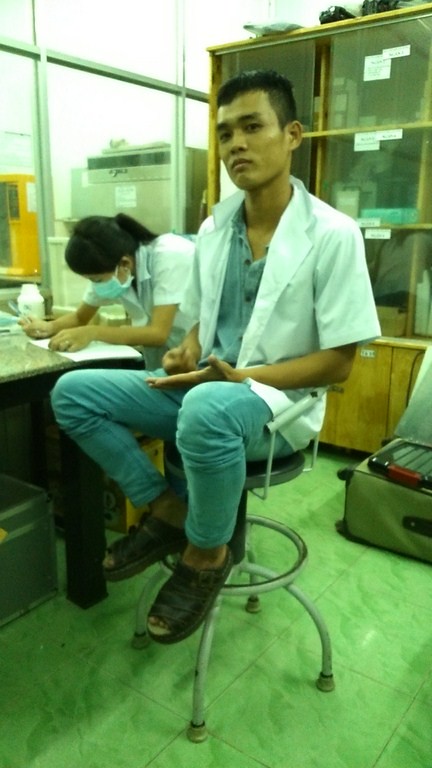This image captures a serious-looking Asian man seated on a white metal stool with four curved legs and a black round seat, positioned inside what appears to be a lab or office environment. He is wearing a short-sleeved white collared shirt over what seems to be blue scrubs or a light denim jumper, and brown open-toe leather sandals. His hair is short and black, with a somewhat faded cut. Directly behind him is a large wooden bookcase with glass doors, containing indistinguishable objects, and adorned with white square cards that have unreadable labels. To the left of the man is an Asian woman, bent over a table, with her black hair tied back in a ponytail and a side-swoop bang. She is wearing a mask and a white lab coat. The setting includes tiled flooring and appears professional, with a grey suitcase also visible in the background, reinforcing the lab or office atmosphere.